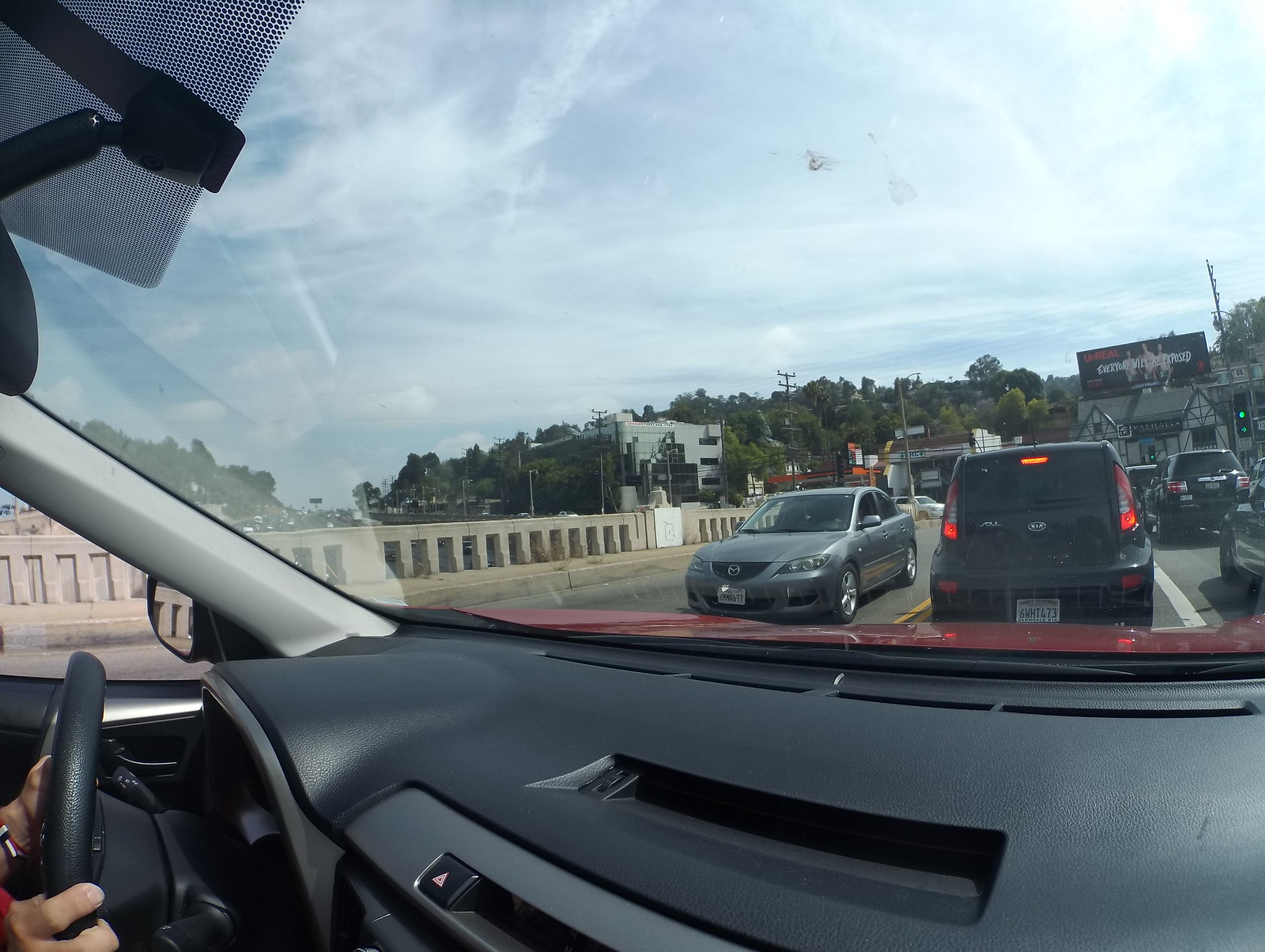A detailed photograph taken from inside a car captures the driver with their hands on the black dashboard steering wheel, adorned with a bracelet on one wrist. Through the windshield, a busy parking lot is visible, populated with various vehicles, including a blackish Kia and a gray car with its headlights off, facing the car. Scattered throughout the parking lot are the partial silhouettes of additional parked cars. In the distance, a green traffic light indicates "go," and behind it stands a large billboard flanked by buildings, one of which appears to be a house or office. Beyond this scene, more structures stretch along the street, and a concrete barrier resembling a highway divider serves as a protective railing to prevent falls from the parking lot.